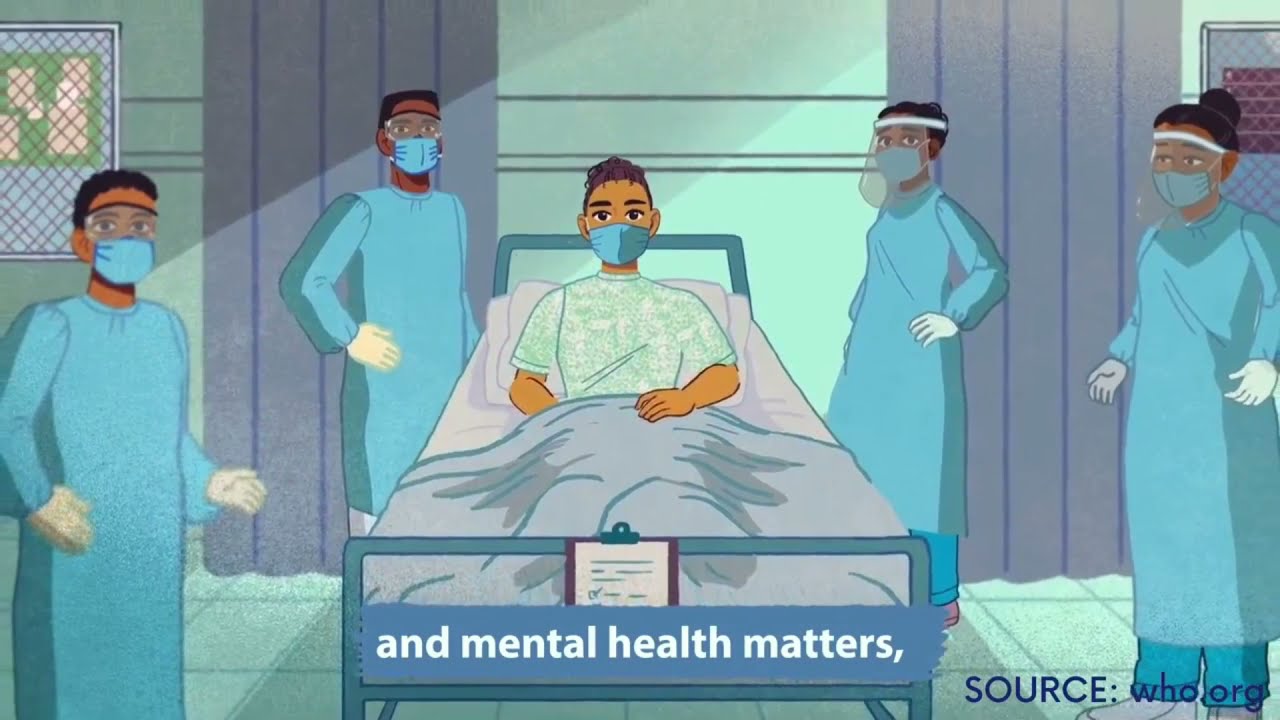In this detailed cartoon illustration set inside a hospital room, a patient with short hair and brown skin sits in a bed covered by a gray blanket. The patient, wearing a green hospital gown and a blue face mask, is surrounded by four doctors. On the left side of the bed are two male doctors, and on the right side are two female doctors, all of African American descent. The doctors are clad in long blue medical aprons, white gloves, face masks, and some also wear extended plastic face shields. The room features a blue-tiled floor and curtained walls with a green bulletin board on one side. A clipboard with writing rests at the patient's feet. The bottom of the image contains the text “Mental Health Matters” in white, and in the bottom right corner, the source “who.org” is indicated in dark blue. The scene is rich with hues of blue, teal, purple, gray, and brown, conveying a message focused on mental health advocacy by who.org.